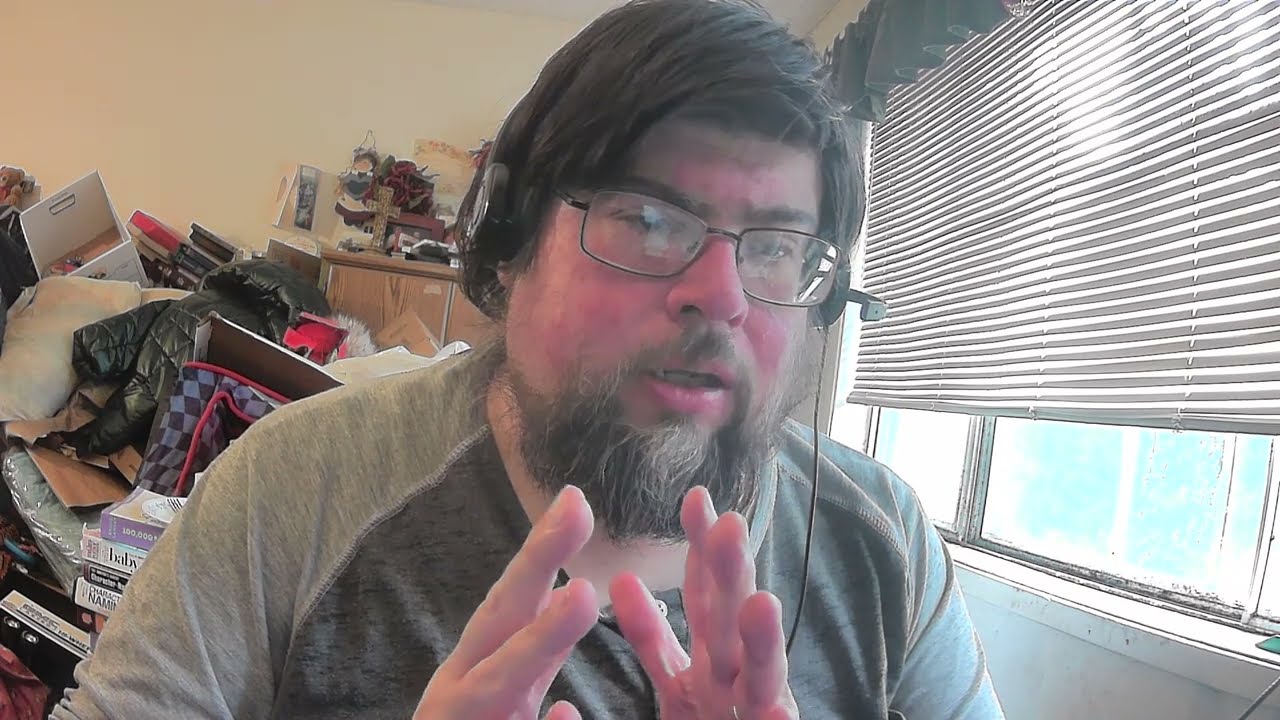This image captures a middle-aged man with thick, dark hair and a beard speckled with gray, engaged in a heated argument. His face is flushed red and his mouth is partially open, revealing slightly crooked teeth. He wears black-framed glasses and a gray shirt, and has a headset on, with the microphone clearly visible. His hands are raised in front of him, palms facing each other, seemingly gesturing as he speaks. Behind him, the scene is cluttered: several books are piled up, a box lies on its side, clothes are strewn about, and a dresser is covered with various items. To his right, a large window with partially open blinds allows sunlight to stream in, highlighting the disarray in the room. A frilly curtain tops the window, adding a touch of detail to the background, which contrasts with the primary focus on the agitated man in the foreground.